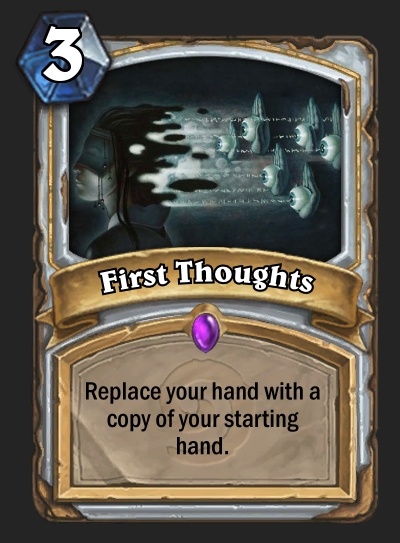The image is of a vertical rectangular game card with a black background and a gold and gray border. In the upper left corner, there's a blue hexagonal gem with a white number "3" on it. The central image depicts an abstract scene with multiple sets of disembodied eyes floating from the right side toward a figure on the left. This figure appears to be a woman's head and neck with black hair, wearing a mask, and facing left. Dotted lines and cloud-like shapes connect the eyes to the figure, conveying thoughts or vision. Across the middle, there's a gold banner displaying the text "First Thoughts" in white. Below this banner, the card contains instructions in a black font: "Replace your hand with a copy of your starting hand." This text is presented within a rounded rectangular area with a purple gem at the top center. The card appears to be part of an unspecified game, with no additional markings or titles indicating the game's name.